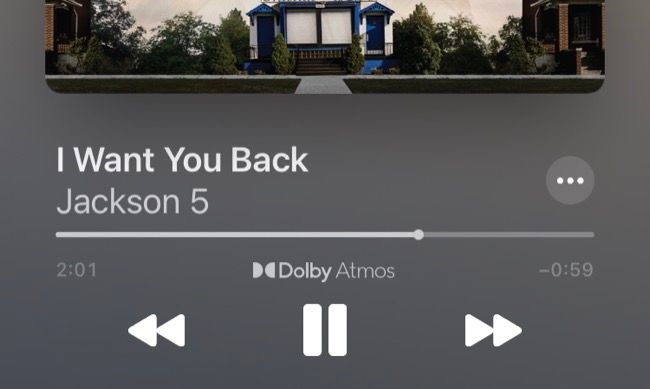This image appears to be a snapshot from a music video, prominently featuring the song "I Want You Back" by the Jackson 5. At the top of the image, there's a horizontal strip displaying a serene scene with trees and a quaint, tiny house in the middle. The house is painted royal blue and has two white windows in the front. A sidewalk extends from the house's entrance, guiding the viewer's eye towards the foreground. The background of the image is set against a deep gray tone, creating a striking contrast with the elements in the scene.

In white text over this background, the title "I Want You Back" and the artist "Jackson 5" are clearly visible. At the end of this text row, there is a gray circle containing three horizontal white dots, suggestive of a menu or options icon in many media players.

Towards the bottom, there's a progress bar indicating the playback status of the video. The bar shows that approximately three-quarters of the song has been played, with a white segment on the left transitioning to a white dot, followed by a gray segment indicating the remaining portion. The elapsed playback time is shown as "2:01," with the Dolby Atmos logo nearby. Additionally, a timer displaying "-0:59" likely indicates the remaining duration of the song. Positioned centrally, control icons for replaying, pausing, and skipping forward are also visible.